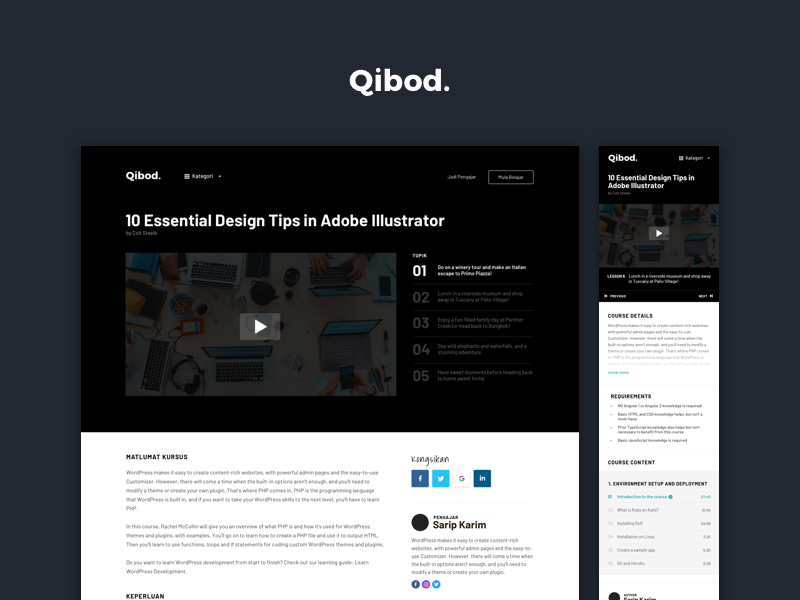In the image, there is a black background with large white text displaying "Q-U-I-B-L-D, Q-B-O-D" at the top. The main focus of the image is centered around a video thumbnail that features the text "Ten Essential Design Tips in Adobe Illustrator." This thumbnail includes an image of a table surrounded by people, many of whom are using laptops. Several hands are visible on the laptops, emphasizing a collaborative or instructional setting. A prominent play button is superimposed over the thumbnail, indicating that it is a video.

Adjacent to the video thumbnail, the text "Number One" alongside some detailed information is also displayed in white. Below this, the numbers two, three, four, and five are listed in gray text. On the right side of the image, "Q-U-I-B-L-D" is reiterated along with "Ten Essential Design Tips in Adobe Illustrator," followed by another thumbnail of the same video featuring a play button. Below this, there are sections labeled "Course Details," "Information," "Requirements," and "Course Content," each accompanied by detailed lists. In the middle of the image, the text "Mat-L-U-M-A-T-K-U-R-S-U-S" is prominently displayed.